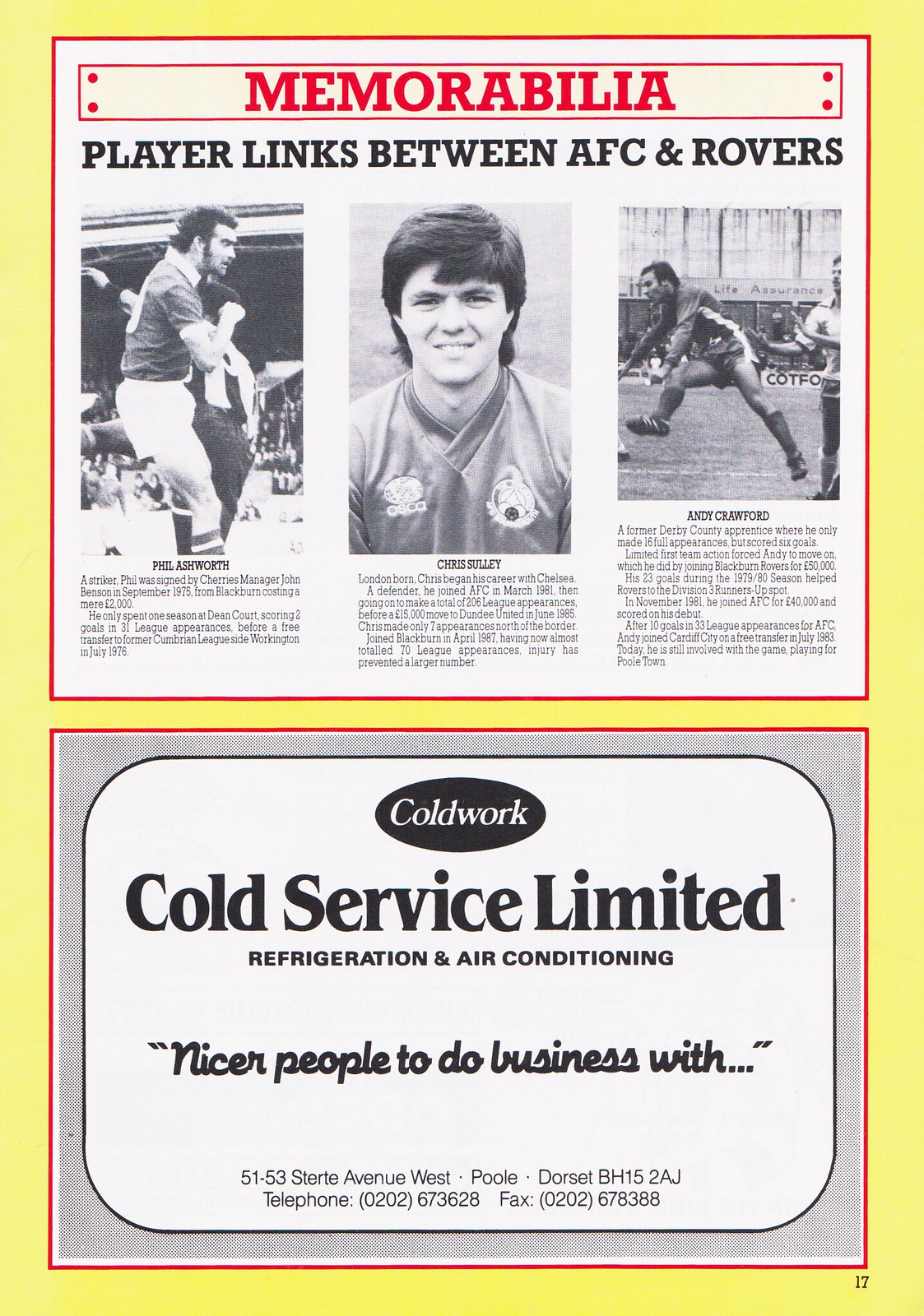This image depicts page 17 of a game day pamphlet or magazine, with a yellow background and a prominent white box bordered in red occupying the top half of the page. Within the white box, the red header text reads "Memorabilia," followed by smaller black text stating "player links between AFC and Rovers." The page features three columns side by side, each containing a photo of a different player. The left photo shows Phil Ashworth, the middle photo features Chris Sully, and the right photo presents Andy Crawford. Below each player's image, their names are written in bold text accompanied by a short biography. Beneath these columns is a red-bordered square advertisement for Cold Work Cold Service Limited, a refrigeration and air conditioning company, with the slogan "nicer people to do business with..." and the address "51-53 Sturt Avenue, West Poole, Dorset BH15 2AJ" along with a contact number.